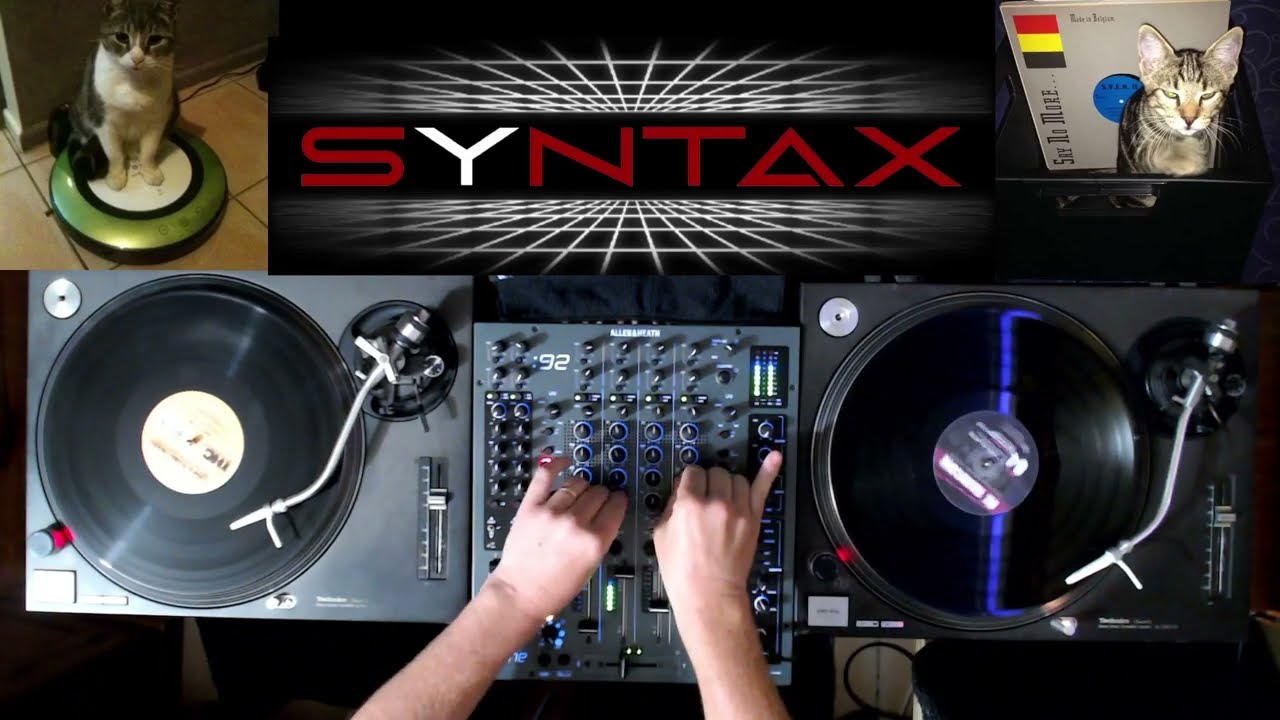In the image, there is an advertisement featuring DJ equipment prominently displayed. The centerpiece is a mixing board with an array of dials and tuner buttons. Flanking the board are two turntables, each actively spinning vinyl records, creating a sense of motion with blue reflections visible on the records. Two pale white hands emerge from the bottom of the image, adjusting the knobs on the mixing board.

Above the equipment, the word "SYNTAX" is illuminated in bold red letters, with the exception of the "Y," which is in white. The letters appear to be connected by a grid-like pattern leading to the word. To the left of the "SYNTAX" logo, a gray and white cat sits atop a robotic vacuum cleaner, resembling a Roomba. To the right, another gray and white cat is positioned in front of a crate of records. This crate bears a sign or flag featuring the colors of the German flag—black, red, and yellow. The overall scene is vividly colorful, featuring hues of black, white, red, blue, green, gray, and tan, enhancing the captivating advertisement likely promoting the DJ brand "SYNTAX."